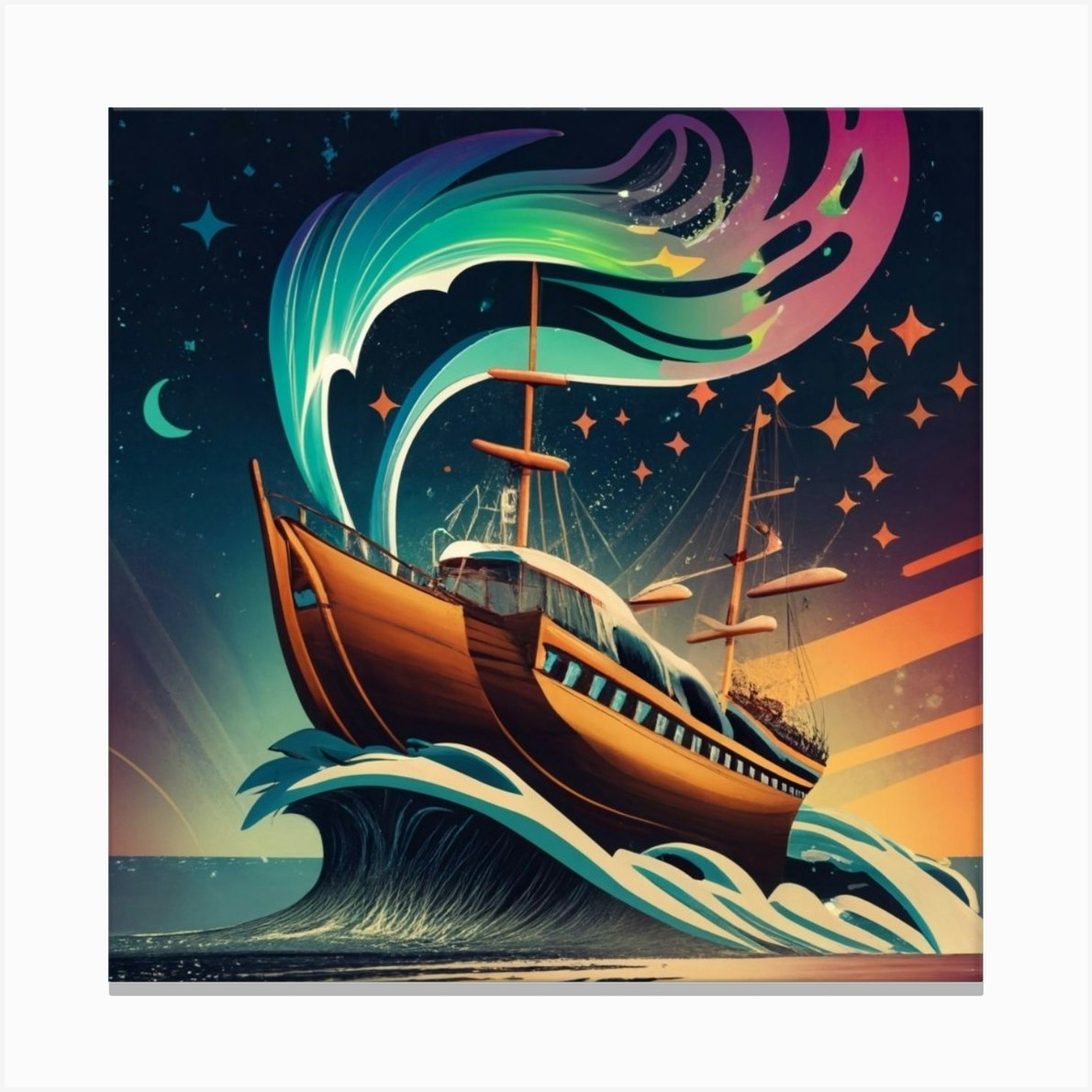This stunning digital illustration features a large, enchanting wooden ship resembling a pirate vessel, captured at the crest of a powerful wave. The ship, with its masts raised but sails tied down, boasts a magical sail adorned with vibrant shades of blue, purple, and pink. The scene is set against a dramatic sky that transitions from a bright, sunset-lit palette of pinks and orange on the right to deep blues and teals on the left, showcasing an ethereal half-moon and a scatter of blue and orange stars. At the bottom left, there's a blend of blues and greens adding to the dreamlike ambiance. The wave, black underneath with a blue and creamy white crest, embraces the ship, directing the viewer’s focus to the colorful matte sail and the wave design emanating from the boat that transitions from blue to green to pink. This image is encased by a white border, adding to its framed, artistic presentation.